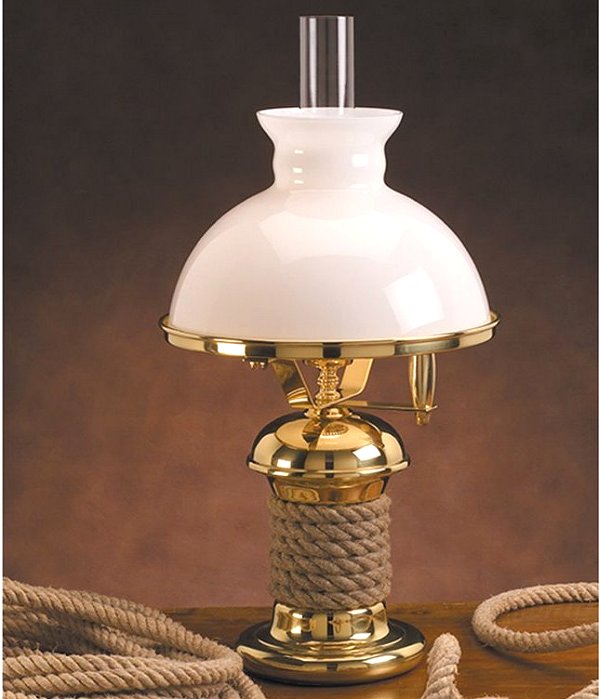The photograph features an intriguing old-fashioned lamp resting on a medium brown wooden table. The backdrop is an ombre of tan to dark brown, giving the setting a rustic feel. The lamp itself stands out with its golden, shiny body, intricately wrapped with a tan rope around the base, making about six tight loops. The base is sturdy, transitioning into a gold stand leading up to a porcelain white dome-shaped lampshade, adorned with a subtle gold trim at its bottom. Emerging from the top of the shade is a clear plastic or glass cylindrical tube, reminiscent of kerosene lamps. Adjacent to the lamp on the table, coil remnants of the same tan rope are thoughtfully placed, adding to the vintage charm of the scene.